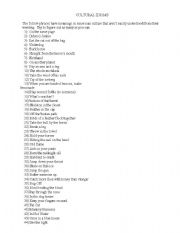This image features a white background with small, black text organized in numbered lines from 1 to 44. Located at the top is a heading, which, despite being slightly blurry, is composed of the same small, black font. Each line from 1 at the top-left corner to 44 at the bottom of the image contains some form of text. Even upon zooming in, both the heading and the individual lines of text remain small and somewhat difficult to read. There are no other colors present in the image, making it a simple monochromatic scheme.